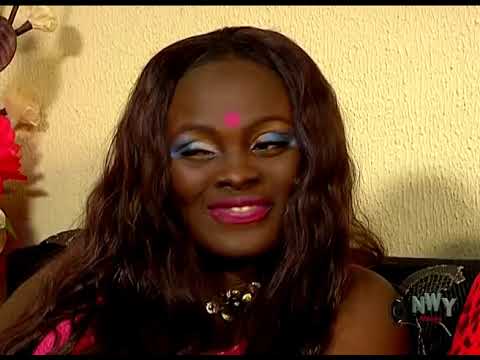The image features a black woman with medium-to-long black hair, seated on a black sofa against a rough-textured yellow wall. She is shown from the armpits up, smiling and looking slightly to her right. She is adorned with striking makeup: bright blue eye shadow accentuated with yellow at the edges, and vibrant pink lipstick. A distinctive pink dot is centered on her forehead between her eyebrows, hinting at cultural significance. She is wearing a shiny golden necklace and possibly a black-and-pink or hot pink shirt, though her bare shoulders suggest the garment may be off-shoulder. The polished frame of the image includes a thin black bar at the top and bottom, with the bottom right corner marked by a gray 3D logo resembling "NWI" or "NWY" over a harp-like symbol.